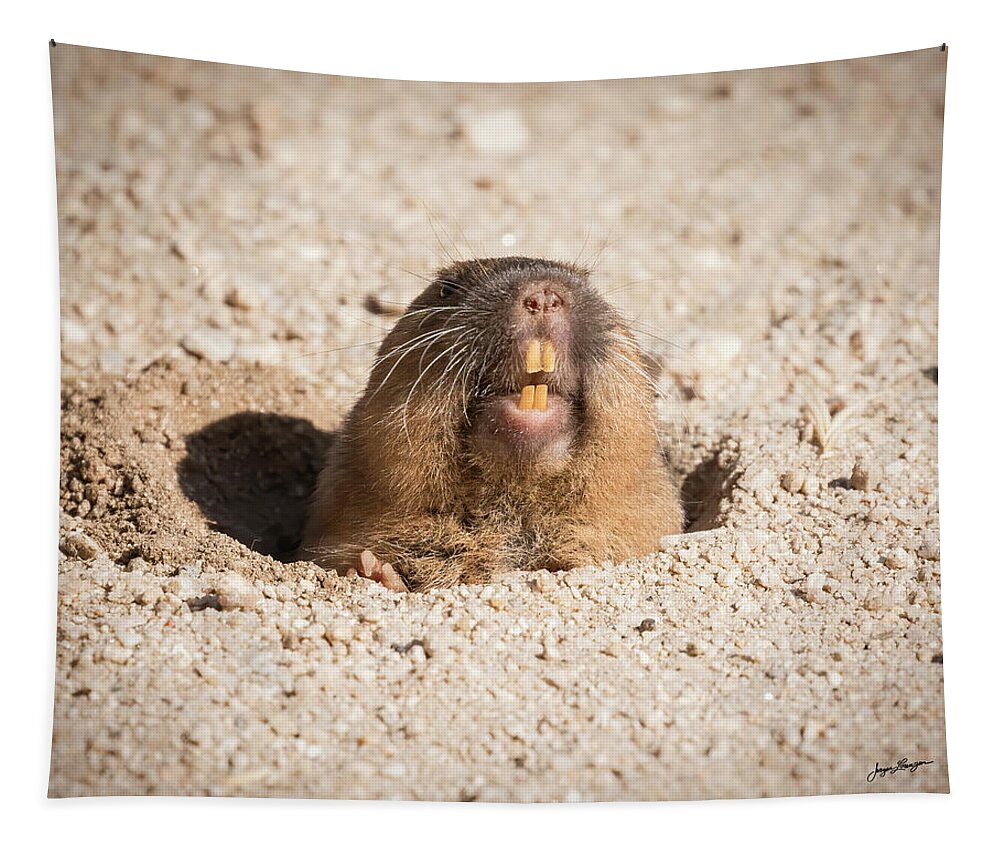This close-up photograph captures a mole emerging from a hole in sandy soil, with its head and shoulders visible. The mole, characterized by thick white-brown fur and large yellowish buck teeth—two at the top and two at the bottom—has its nose and whiskers prominently displayed, with whiskers extending symmetrically around its snout. One of its eyes is visible while the creature’s sharp claws are evident on a paw resting on the hole’s edge. The sandy soil is mostly a gray and light brown mix, with noticeable granularity and varying shades around the mole. In the lower left corner, there is a cursive signature in black, likely the photographer's, which appears to read "Sagni Lananga," but is somewhat difficult to decipher. The scene is brightly lit, suggesting the picture was taken during daylight hours, and the background is slightly blurred, drawing attention to the detailed features of the mole in the foreground.